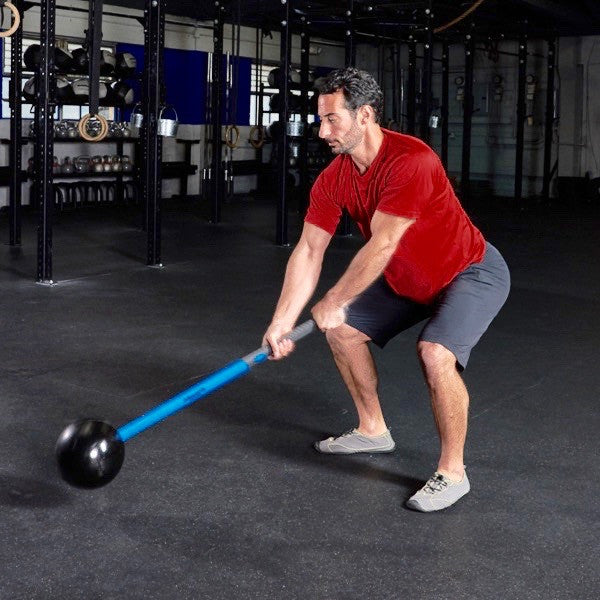The color photograph captures a man exercising in a gym, which appears to be in a garage or industrial-style building. The man has dark, short hair and some facial hair, and is wearing a short-sleeved red shirt, gray shorts, and gray sneakers. He is facing left while squatting down, holding a unique exercise tool in both hands. This tool consists of a long blue rod with a gray handle and a solid black ball at the end, resembling a weighted sledgehammer. He appears to be performing a CrossFit-style workout, potentially preparing to swing the tool down to hit the floor. The gray floor beneath him and the dark background are contrasted by the lighting focused on him. Behind him, various gym equipment such as pull-up bars, kettlebells, and gymnastics rings are visible, along with shelving units holding additional sports gear. The setting and the man's posture suggest an intense workout session amidst a well-equipped gym environment.